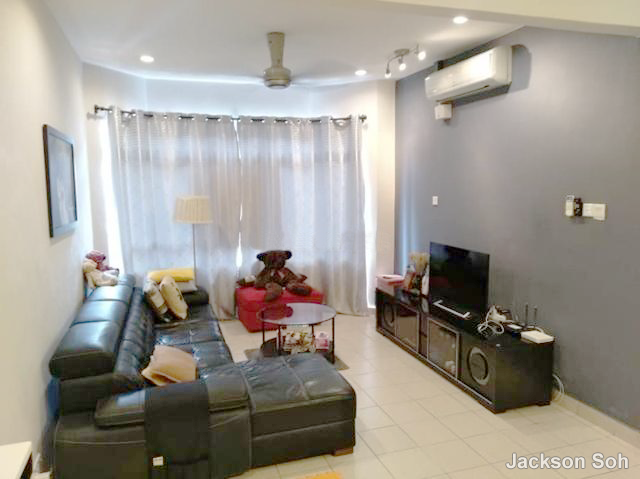In this image, we see a cozy yet modern small living room, characterized by its light beige, square tile flooring. The left wall is painted an off-white color, while the ceiling is a brighter white, creating a fresh and airy atmosphere. The right wall stands out with its light gray hue. Mounted near the ceiling on the right side is a white heat pump, enhancing the room's comfort.

Illuminating the room, recessed pot lights are complemented by an off-white ceiling fan, which gently rotates its blades. A brown curtain rod stretches across a window, adorned with white curtains that softens the room's ambiance.

To the left, there is a gray picture frame hung on the wall. Below the window, a stylish white-shaded lamp with a silver pole adds a modern touch. Adjacent to it, a grayish-green leather couch with beige pillows offers comfortable seating. On the couch, a white and a pink stuffed animal lean against the wall, adding a whimsical note. Leaning against the window curtain is a brown teddy bear sitting on a red cushion.

A glass-topped coffee table with black legs occupies the center of the room, while to the right, a black small table stand supports a flat-screen TV and a white Wi-Fi box. Additionally, a gray plush teddy bear sits to the left. Two black speakers flank glass doors, framing the living space.

In the bottom right corner, in white font, the text "Jackson's Sew" is subtly displayed, adding a personalized touch to this inviting living area.